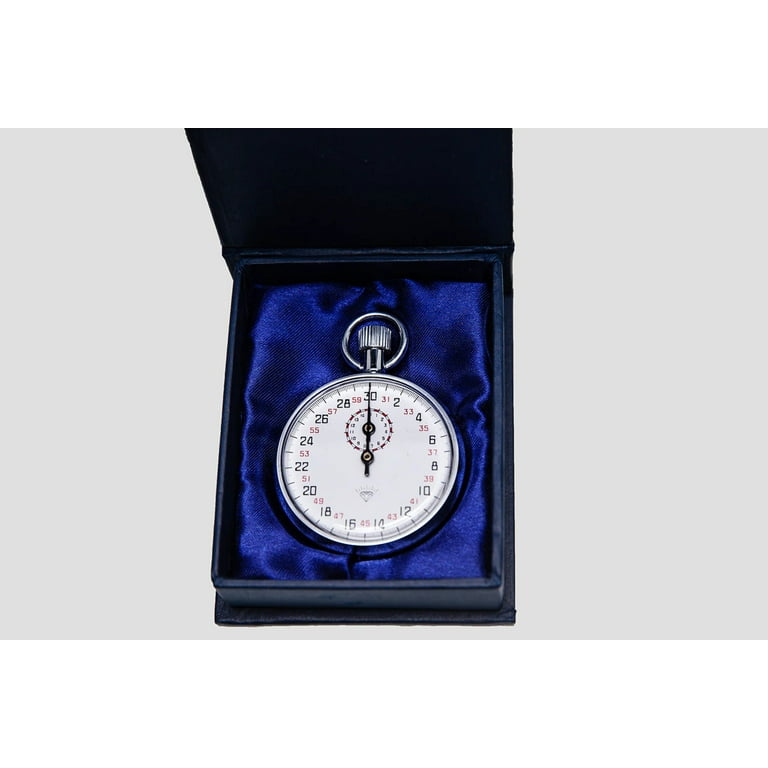The image depicts a high-end stopwatch set within an ornate black case, adorned with a luxurious, royal blue velvet or satin interior. The stopwatch itself features a silver exterior and a white face with black primary numbers and red secondary numbers around its circumference. Positioned centrally within the case, the stopwatch displays its hands pointing to the 30 mark at the top. In addition to its elegant silver loop and a knob at the top for operation, the watch includes a smaller sub-dial just below the main hands. The case is open, with its top section exiting the frame, and sits against a plain light gray background, suggesting a minimalistic surface that emphasizes the watch's sophistication.